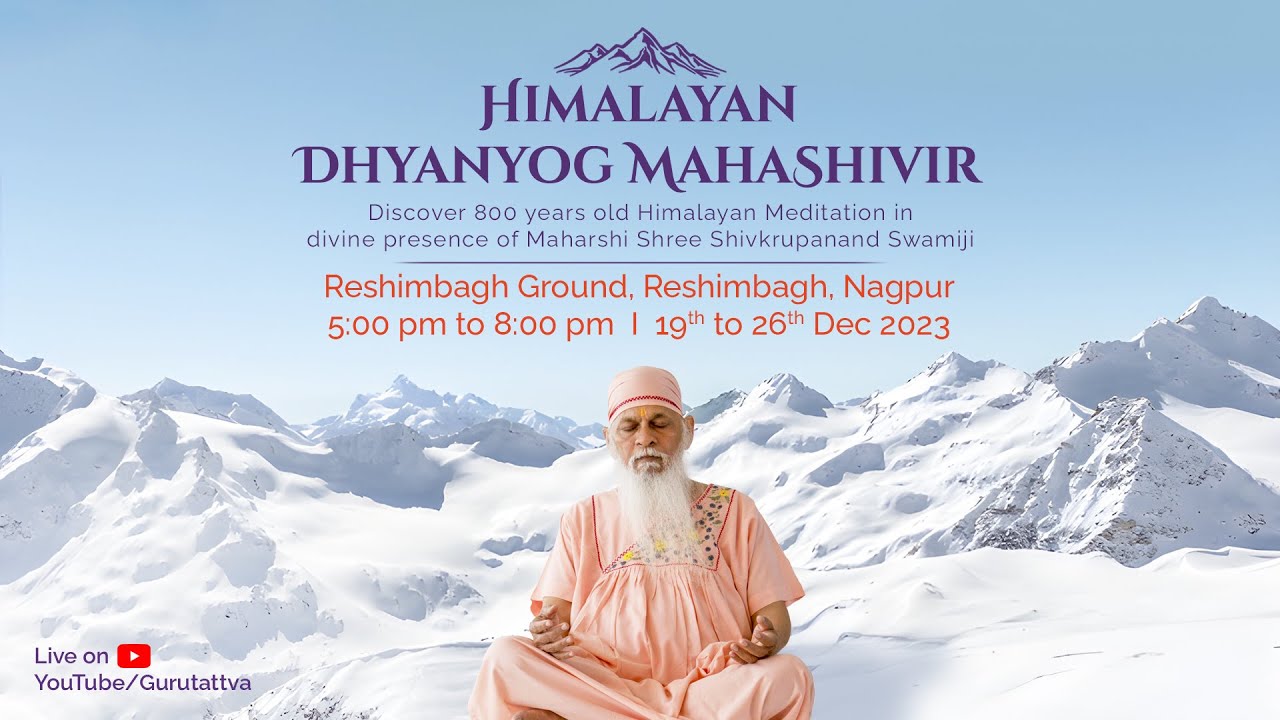This image is a detailed poster advertising a Himalayan meditation event, titled "Himalayan Dhyan Yog Mahashivir." The event promises an exploration of an 800-year-old Himalayan meditation practice and the divine presence of Maharshi Shri Shivkrupanad Swamiji. The event will take place at Rishin Bagh Ground in Nagpur from December 19th to 26th, 2023, between 5 p.m. to 8 p.m. daily. The poster also highlights that the event will be streamed live on YouTube via the channel "Guru Tattva Tattva." Dominating the center of the poster is an image of Maharshi Shri Shivkrupanad Swamiji, portrayed as an elderly man with a white beard. He is dressed in a pink robe and matching turban, seated in a meditative pose with his eyes closed and hands raised on a snowy mountaintop, which appears to be digitally rendered. The vibrant hues of purple and orange used in the text contrast against the serene, snowy Himalayas background, further emphasizing the spiritual and ethereal nature of the event.